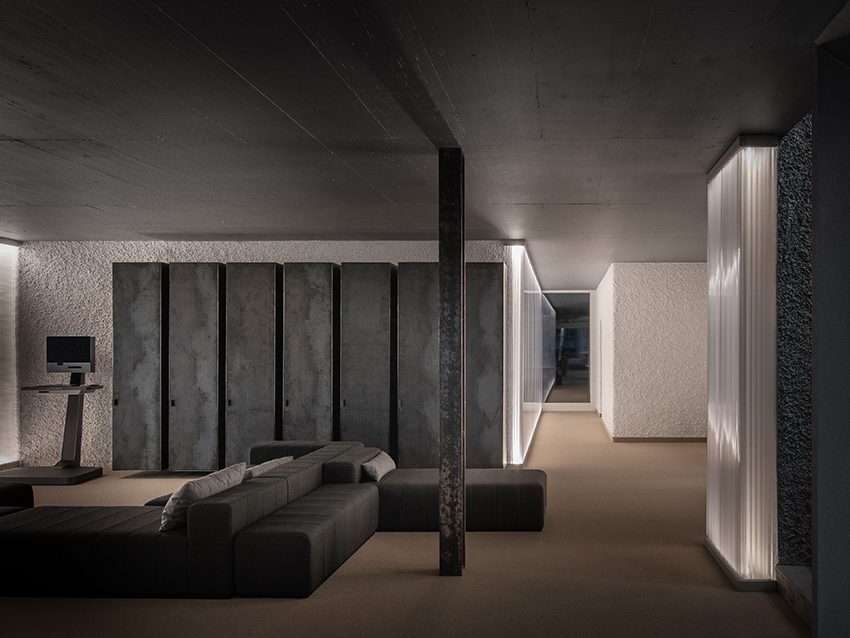The image depicts a modern, industrial-style interior space that could serve as either a home or an office. Dominated by a palette of gray, brown, and white, the decor features dark gray, rectangular sofas from Ikea, arranged in back-to-back L-shapes. These sofas are sparsely adorned with light gray pillows, creating a rather hard and uncomfortable seating area. A prominent metal column stands in the middle of the room, adding to the industrial feel. 

The left side of the room houses a standing desk with a computer monitor, reminiscent of the roll-around stations used in hospitals. Along the left wall, there's a row of metal lockers, enhancing the utilitarian aesthetic. The room also features decorative wall lights, with dim lighting providing a subdued ambiance. The ceiling, gray in color, sits above walls that have a textured, popcorn finish.

A long hallway extends from the space, ending in what appears to be a mirror, while the right side of the room is lit by full wall lights. The ceiling is relatively tall, contributing to the airy, spacious feel of the room. Overall, the design is sleek and modern, yet retains a somewhat cold and uninviting atmosphere due to the stark, minimalistic furnishings and the muted color scheme.